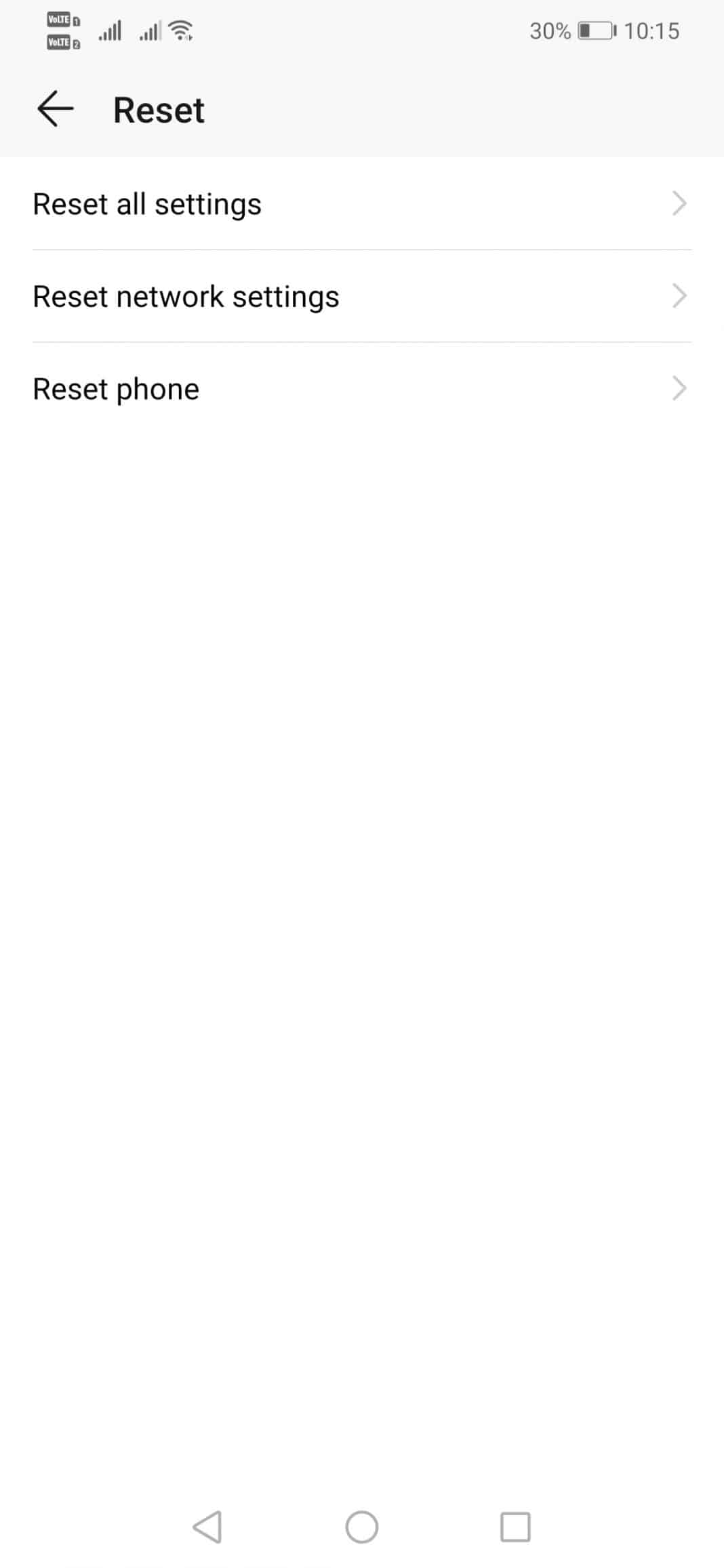A mobile screenshot from an Android device displaying the reset settings menu. The device interface includes navigation buttons at the bottom: a triangle on the left, a circle in the center, and a square on the right. At the top of the screen, the status bar shows two distinct cell network connections, each indicating LTE with one network having five bars and the other four. The Wi-Fi signal is full, the battery level is at 30%, and the time is 10:15. 

A significant portion of the image, around 75%, is blank white space. Positioned beneath the notification icons is a black arrow pointing to the left next to the word “Reset.” The screen displays three reset options: "Reset All Settings,” "Reset Network Settings,” and "Reset Phone," each separated by a pale gray divider and accompanied by a gray arrow pointing to the right, suggesting further settings available. This screenshot likely illustrates how to access the reset options on an Android phone.